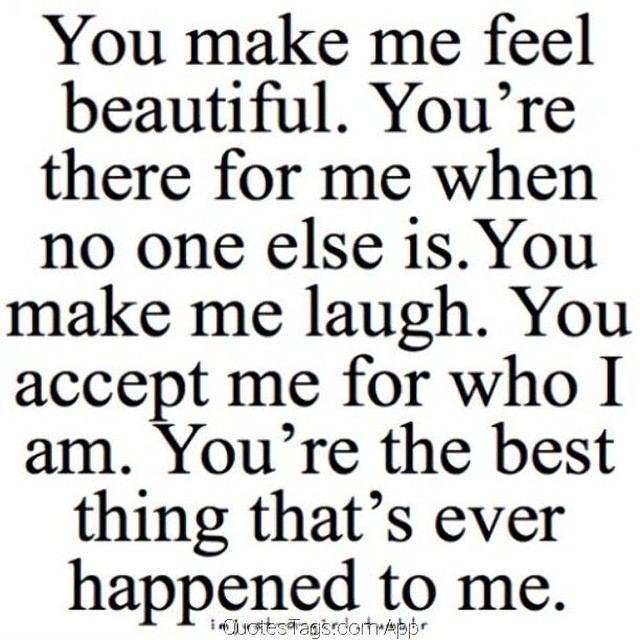This image features a text block on a stark white background, with the message written in large, bold black letters. The heartfelt paragraph reads: "You make me feel beautiful. You're there for me when no one else is. You make me laugh. You accept me for who I am. You're the best thing that's ever happened to me." The text spans nine horizontal lines, with each line containing four to five words due to the large font size. At the very bottom in smaller black letters, it reads, "quotestext.com app."